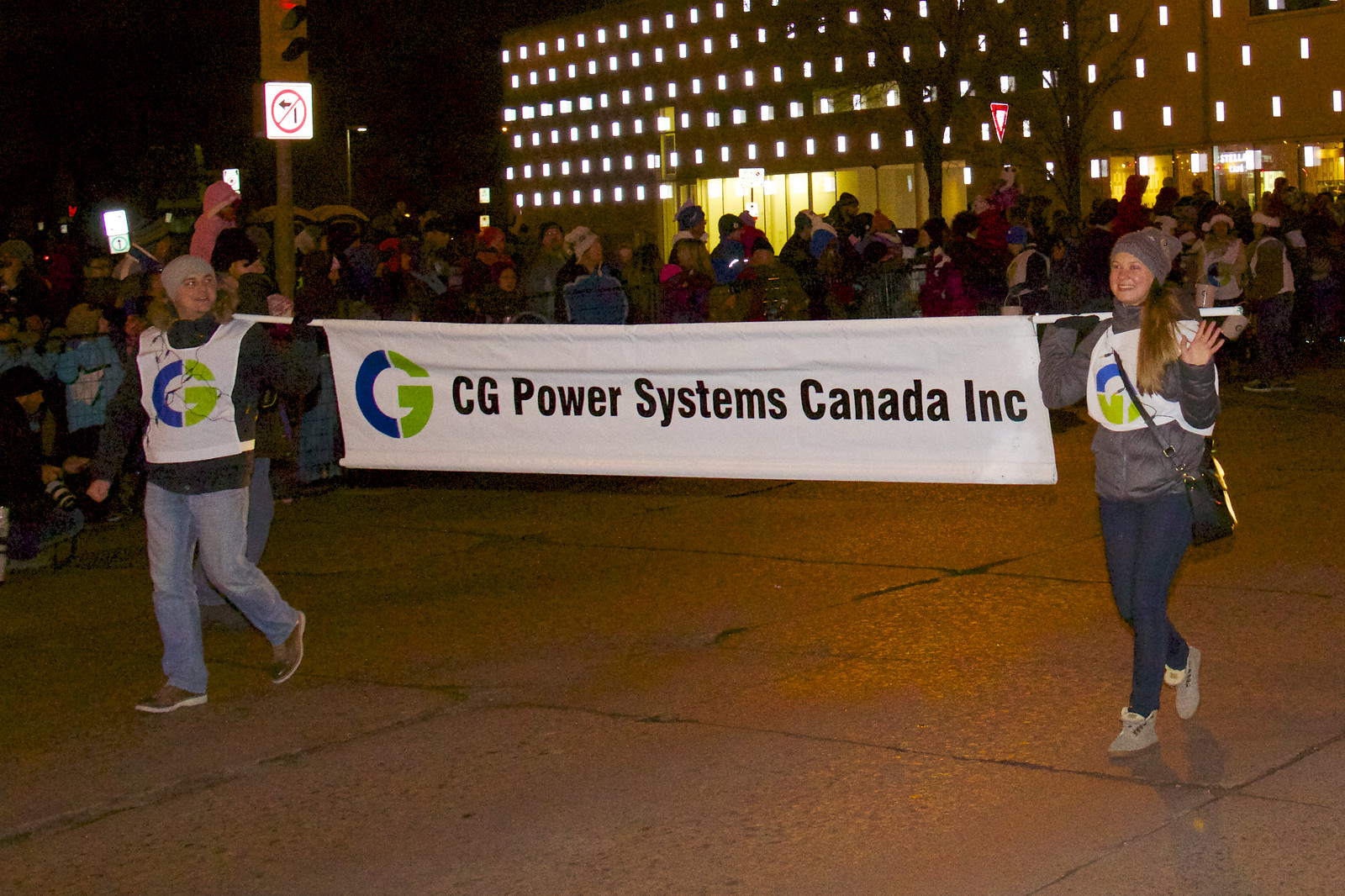The nighttime photograph captures a scene from a parade featuring two women as the main focus, each holding one end of a long white PVC pole that stretches between them. They are carrying a horizontal vinyl banner that reads "CG Power Systems Canada Incorporated" in black text, accompanied by a blue and green "G" logo. The woman on the left wears a grey zip-up hoodie, blue pants, grey shoes, a black purse, and a grey beanie, and she gazes at the woman on the right. The woman on the right, dressed in jeans, brown shoes, a black zip-up hoodie, and a light grey beanie, smiles and waves at the camera. In the background, a large crowd of spectators, clad in jackets and beanies, suggests a cold night. The crowd is somewhat indistinct due to the darkness, but the illuminated traffic lights, signs, and numerous warmly lit rectangular windows of a very long building in the background add ambiance to the scene.